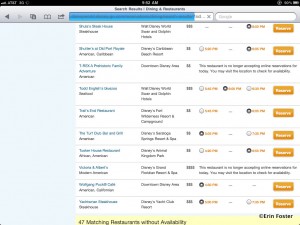The image is a small, heavily cropped screenshot, likely taken from a tablet device. It features a thin black bar across the top. In the upper left corner, there are some white icons or text. The center displays an unreadable time stamp, indicating it is sometime in the p.m. The upper right corner shows a battery symbol along with additional icons. Below this, a gray section includes a bar with a back button and other icons on the left side. The center of this bar contains an address bar, while the right has a search bar. Further down the image, on the left side, there is a blank bluish-gray colored box. The center section features text displayed on a white background, with yellowish-orange buttons aligned on the far right side of each text section, suggesting these could be related to items or options.